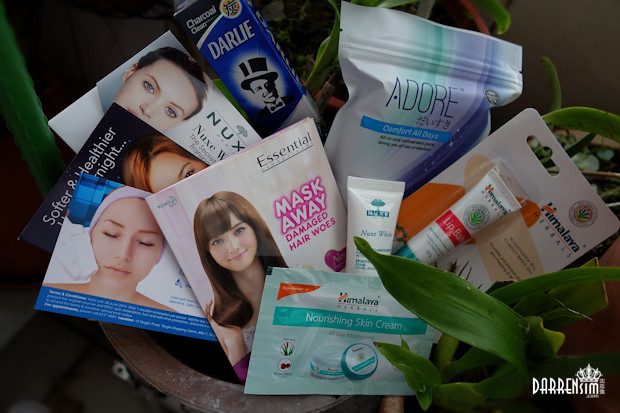The image showcases a variety of hair and personal care products arranged in a visually appealing manner. In the bottom right corner, white text reads "Darren Sim." Surrounding the text are several green leaves and plants, adding a touch of natural elegance to the composition. Central to the image is a basket filled with various hair masks and treatments labeled "Mask Away," each featuring illustrations of faces indulging in a spa-like experience. 

In the top right corner, an unopened package of "Malaya Herbals Lip Balm" stands prominently, suggesting the product's pristine condition. Beside it, there's a package labeled "Adore Comfort All Days" and another product named "Charcoal Clean Darlie," which features the image of a man in a top hat against a blue background. Additionally, the phrase "Essential Mask Away Damaged Hair Woes" is visible near an image of an Asian woman with brown hair and bangs, who embodies the promise of the hair care products on display.